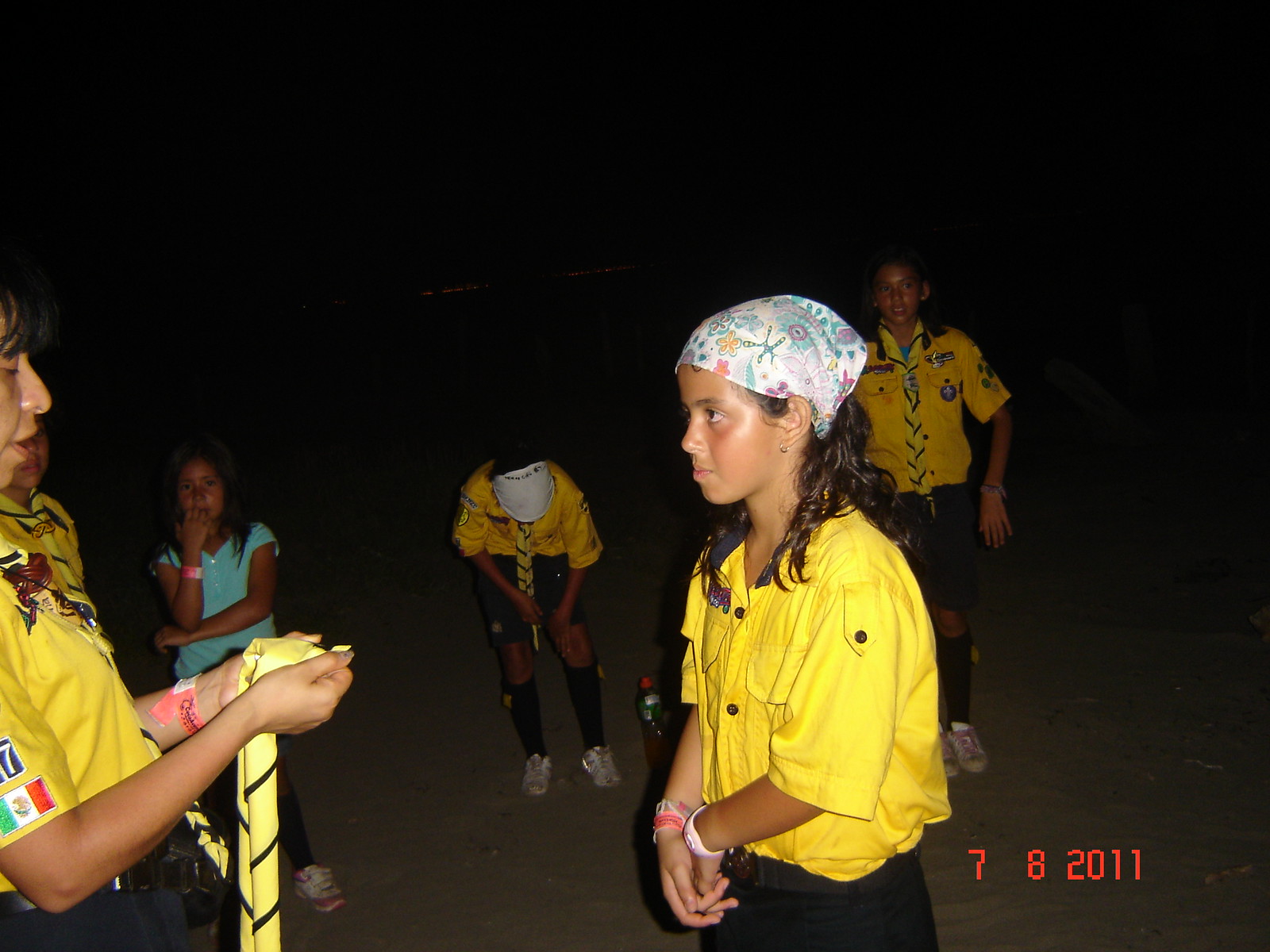In this photograph, taken from an old-timey film camera with a visible date of 7-8-2011 in red digital pattern in the bottom right corner, we see a scout troop standing in the sand during nighttime. The central focus is on a young girl with a white bandana featuring a paisley pattern in teal, pink, and yellow. She has brown hair and wears a bright yellow button-down shirt with no patches, black pants, and a pink bracelet. She stands with her hands crossed in front of her, receiving a yellow and blue tie from an older woman. The older woman, also wearing a bright yellow shirt adorned with two patches—a Mexican flag and a blue patch with white numbers—and black pants, is looking down at the tie she is presenting. In the background, two other scouts in yellow shirts with the same blue and yellow ties are visible; one is leaning down scratching her legs, while the other stares at the camera. Additionally, to the left, a young girl in a bright blue shirt is seen chewing on her fingers. The scene is primarily dark, highlighting the group against the night backdrop.